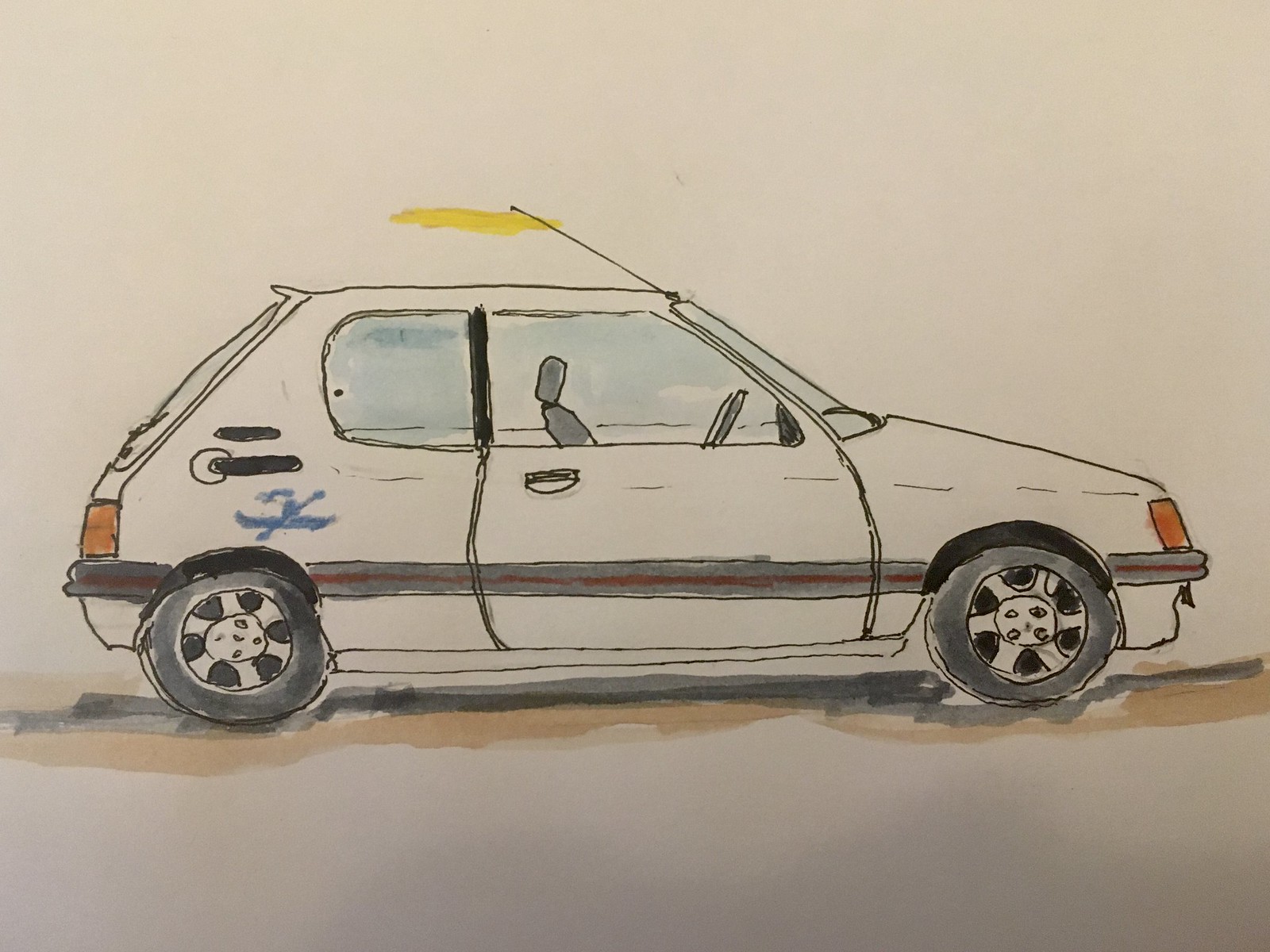A detailed sketch of a white hatchback car, drawn on an off-white beige paper, prominently features the vehicle designed for racing. The car sports a yellow flag protruding from the top of the windshield and a distinctive blue symbol depicting a person in a canoe on the rear. A continuous gray stripe runs from the hood to the trunk, adding to its sleek appearance. The car is elevated by gray tires with white hubcaps and rests on a lightly shaded gray-brown surface. The orange head and tail lights provide a vivid contrast against the white body. Visible through the windows, the interior reveals the seat and steering wheel, indicating that the car is unoccupied.